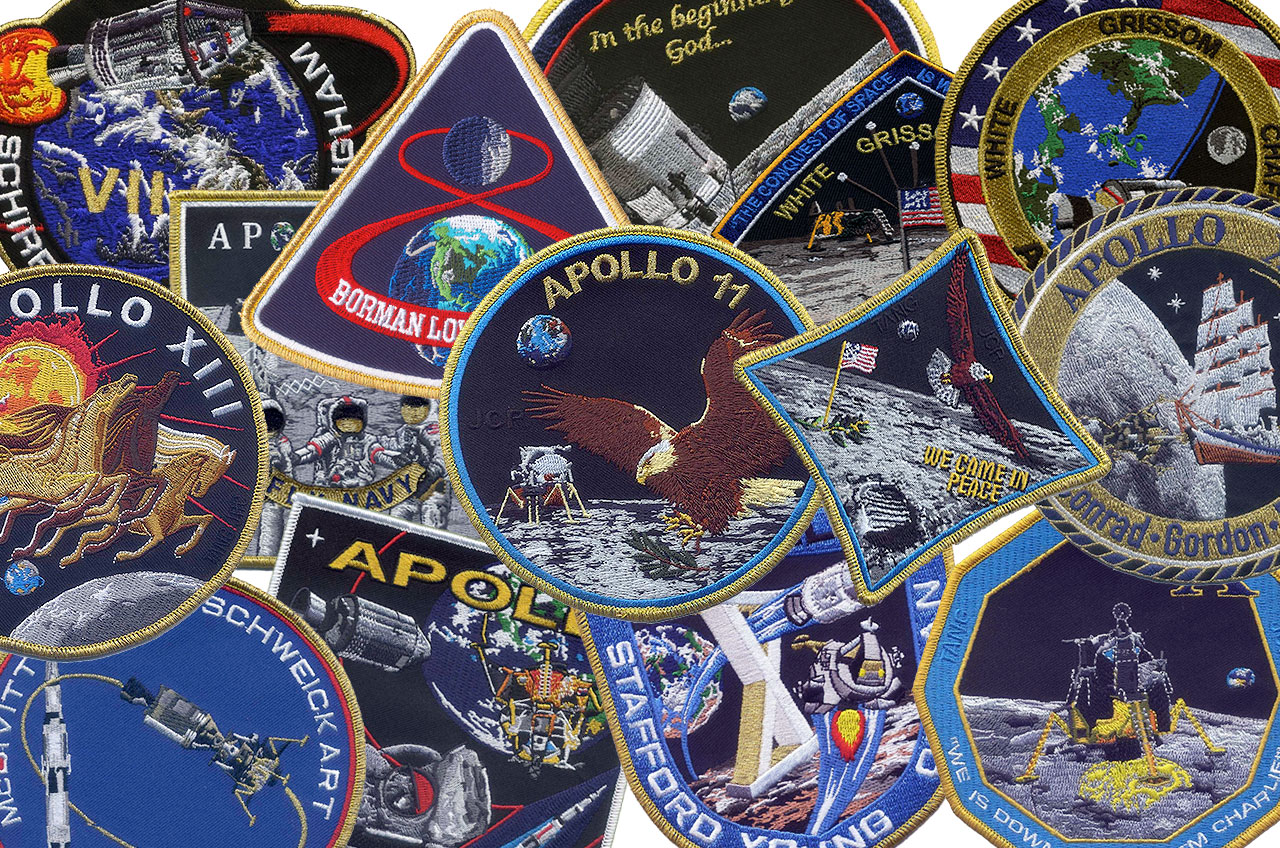The photograph showcases an assortment of approximately 15 NASA mission patches, predominantly from the Apollo space missions, intricately arranged and overlapping against what appears to be a white background, possibly a table. Central to the image is a mostly visible Apollo 11 patch featuring the iconic lunar surface with an eagle landing, Earth in the background, and the lunar module to the left. Adjacent to it, on the right, is a patch with a similar lunar surface, an American flag, and the inscription, "We came in peace." Among the varied patches, there are different shapes including circles, triangles, diamond-shaped, and irregular forms. Visible are patches related to Apollo 13, depicted with horses pulling the sun; Apollo missions with phrases such as "White Grissom" and "Stafford Young;" and one with a red numeral eight encircling Earth and the moon. Despite overlapping, distinct designs like a sailboat, a bald eagle, and a rocket with flames are discernible. The diverse array of emblems stacks densely, emphasizing the rich history of NASA's space expeditions.